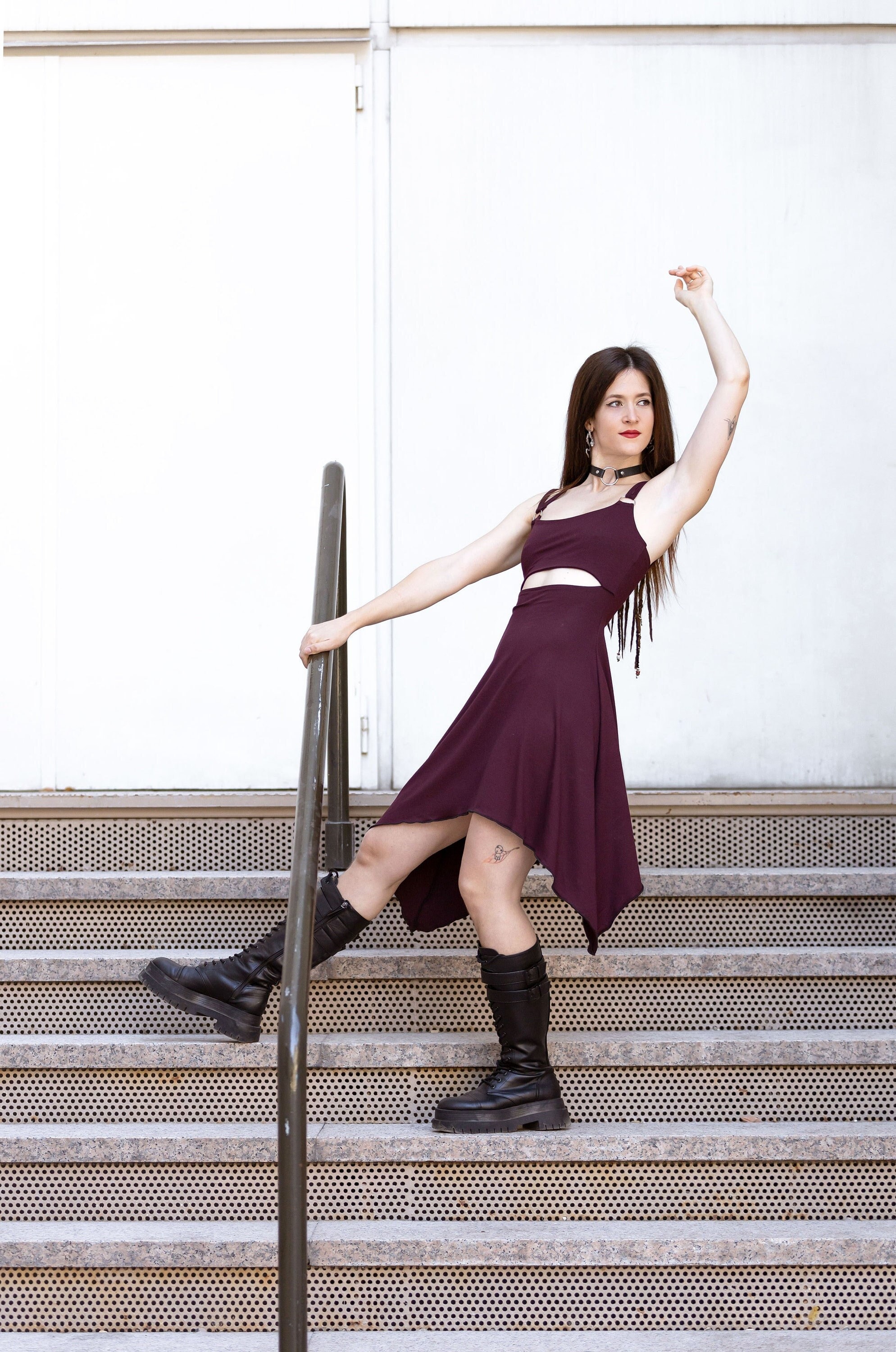In this detailed color image, a woman is striking a dynamic pose on a set of tan, beige-gray stairs that have solid tops and perforated, mesh-covered bottoms. A brown pipe serves as a handrail running down the left side of the stairs, which she holds with her right hand. The woman is positioned in a semi-side profile with her right arm extended above her head, gazing away from the camera. Her right leg is outstretched while she balances on her left leg, creating an upside-down V-shape with her legs. She has dark, straight hair, light skin, and is adorned with red lipstick, silver earrings, and a black and silver metallic choker necklace. She wears a sleeveless, wine-red dress featuring a strappy design with a cutout in the midriff and a handkerchief-style hem that flows to her knees. Complementing her dress, she's wearing black leather combat boots. A small tattoo is visible near her left kneecap. The background is a plain white wall, possibly the exterior of a building, with a white door partially visible.